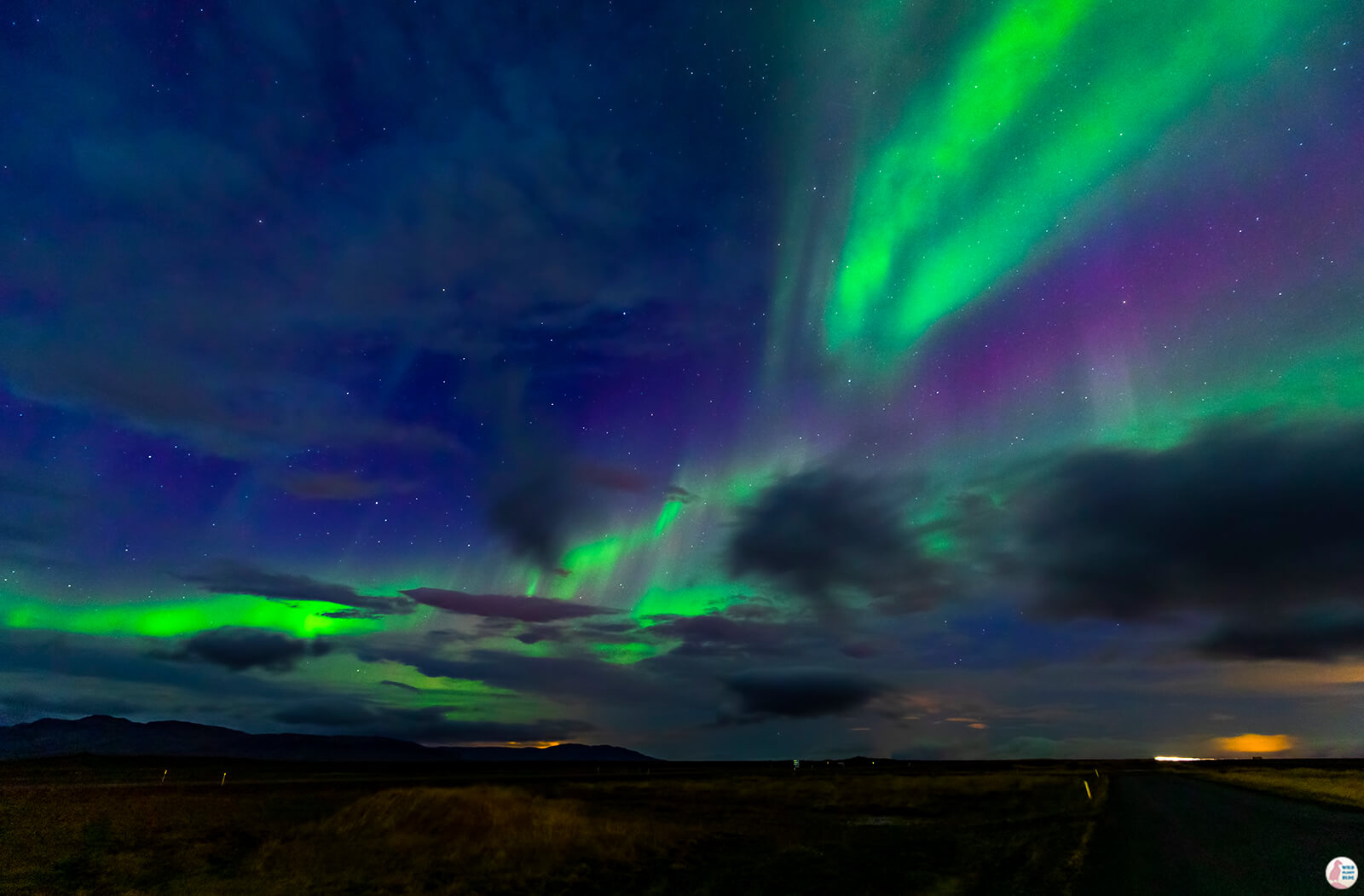This digital image captures a mesmerizing view of the Northern Lights in a rural, likely northern, countryside. Dominating the upper seven-eighths of the frame, the night sky is a dark blue canvas sprinkled with stars, suggesting a long-exposure photograph. The vibrant auroras paint the sky with dazzling streaks of bright green, purple, magenta tones, and hints of light blue and orange. These colors swirl artistically, creating a magical, almost dreamlike atmosphere. Below, a light tan brush indicative of mountains or ground structures frames the scene, with faint shapes of what appears to be farmhouses and a road visible towards the bottom right, softly illuminated by orange lights. The presence of some clouds adds depth, yet the Northern Lights pierce through, maintaining their ethereal glow and enhancing the image's enchanting aura.